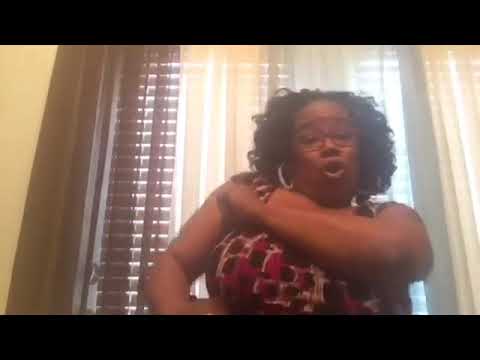This slightly blurry image appears to be a still from a video or a captured moment of an African-American woman positioned from the waist up. She has dark, curly hair that falls to her shoulders and is wearing glasses. Her attire is a red, black, and white sleeveless top, complemented by hoop earrings. 

The woman, possibly in the midst of a dance or a lively expression, has her left arm bent and fist balled up in front of her, while her right arm is caught in motion, possibly coming around her waist. Her mouth is open as if she is singing or passionately speaking. She is positioned against a window with brown wooden borders, from which natural light streams in, partially blocked by wooden cloth blinds and white sheer curtains. The background wall appears to be off-white or beige. The image is framed with thin black rectangles at the top and bottom, possibly suggesting it is a screenshot from a video, likely for YouTube or an instructional dance video. The scene conveys an energetic and expressive moment as the woman engages with her unseen audience.